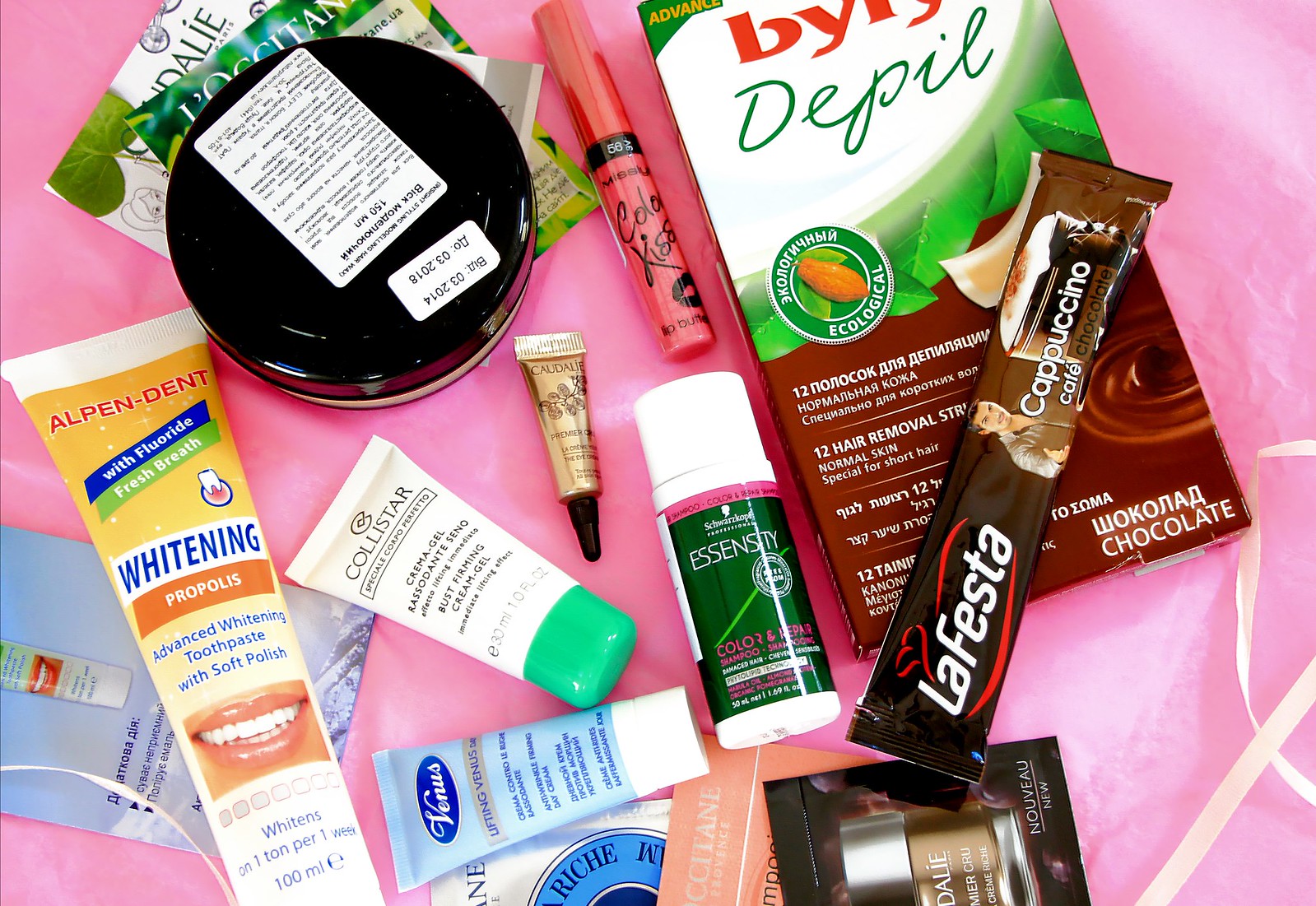This indoor color photograph features a meticulously arranged collection of various objects placed on a vibrant pink cloth. The scene is brightly lit, ensuring each item is in sharp focus. 

Beginning from the upper left corner, a circular object with a glossy black finish, approximately three inches in diameter, is adorned with a white rectangular label. This object is positioned atop a series of rectangular white and green advertisements. Centered in the composition is a rectangular tube of pink lip gloss featuring black lettering. To the right of this, occupying a significant portion of the right side, is a large rectangular box of chocolates. The chocolate box showcases a white label on the upper section and a green one on the lower section, with text in what appears to be Russian.

Diagonally crossing the box of chocolates from the bottom center to the upper right is a thin, rectangular candy bar, approximately an inch and a half wide and six inches long. Its label prominently displays the words "Cappuccino Cafe" written vertically. 

In the center-lower part of the image is a small rectangular beauty product container with a green label and white print. This container, with a white cap, measures about an inch in diameter and three inches in length. Just to the left of this is a small golden tube, about half an inch wide and two and a half inches long, with a black cap oriented downwards. 

Below these items, another tube is situated, wider at the base and becoming cylindrical at the top with a green cap. This tube, inscribed with black lettering indicating it is a bust firming cream, lies nearly horizontal. 

In the lower left corner, an advertisement for a whitening product is visible next to the actual product tube, which extends diagonally from the left and exits the frame at the bottom. This tube, featuring a yellow label with blue lettering that says "whitening," also displays an image of a smiling person's teeth towards the lower part of the label.

Along the bottom edge, several perfume cards in shades of orange and brown are scattered. Additionally, another almost horizontal tube is found here—a blue container labeled "lifting Venus" with blue lettering and a white cap.

The entire collection comprises beauty products, teeth whitening items, and chocolates, each meticulously placed to create a visually engaging layout.